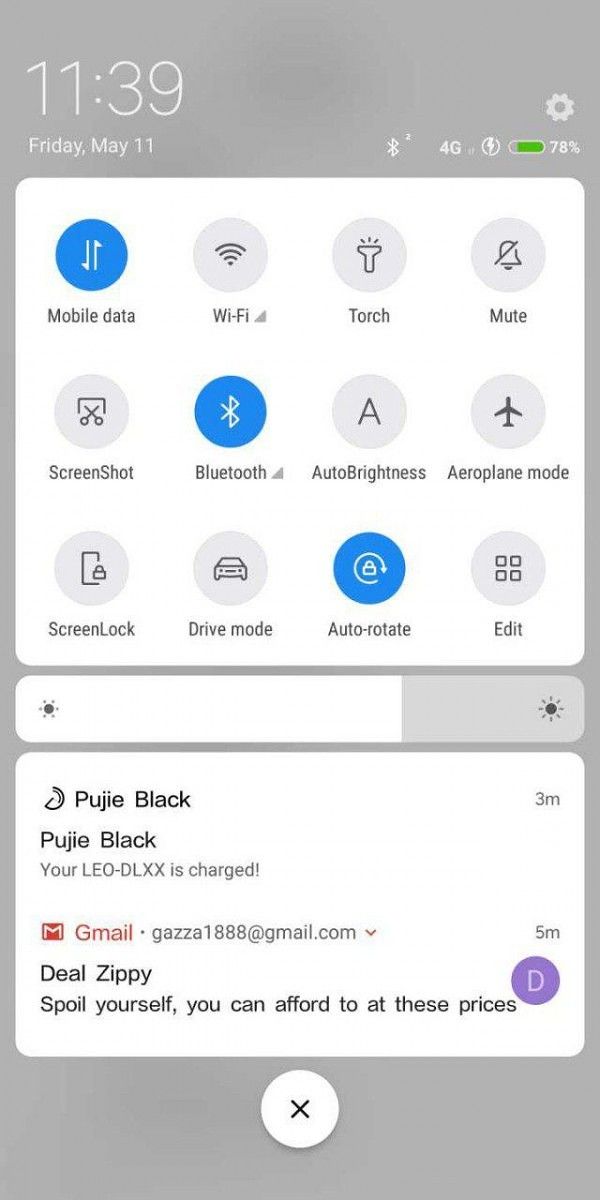This image captures the home screen of a smartphone, showcasing various interface elements. At the top of the screen, the status bar displays the time as 11:39 AM on Friday, May 11th. The status bar also includes several icons indicating the active functions: mobile data, WiFi, Bluetooth, and auto-rotate, each illuminated in blue to signify they are enabled. 

Directly below the time and status icons, there are several quick-access buttons for various features: mobile data, WiFi, torch, mute, screenshot, Bluetooth, auto-brightness, airplane mode, screen lock, drive mode, auto-rotate, and an option to edit these buttons. 

In the lower section of the screen, the text "Poojie Black" is prominently displayed twice. Additionally, the message "your LLDLXX is charged" appears, indicating the device's current charging status. The overall interface is clean and well-organized, providing easy access to essential functions and clear information about the device.